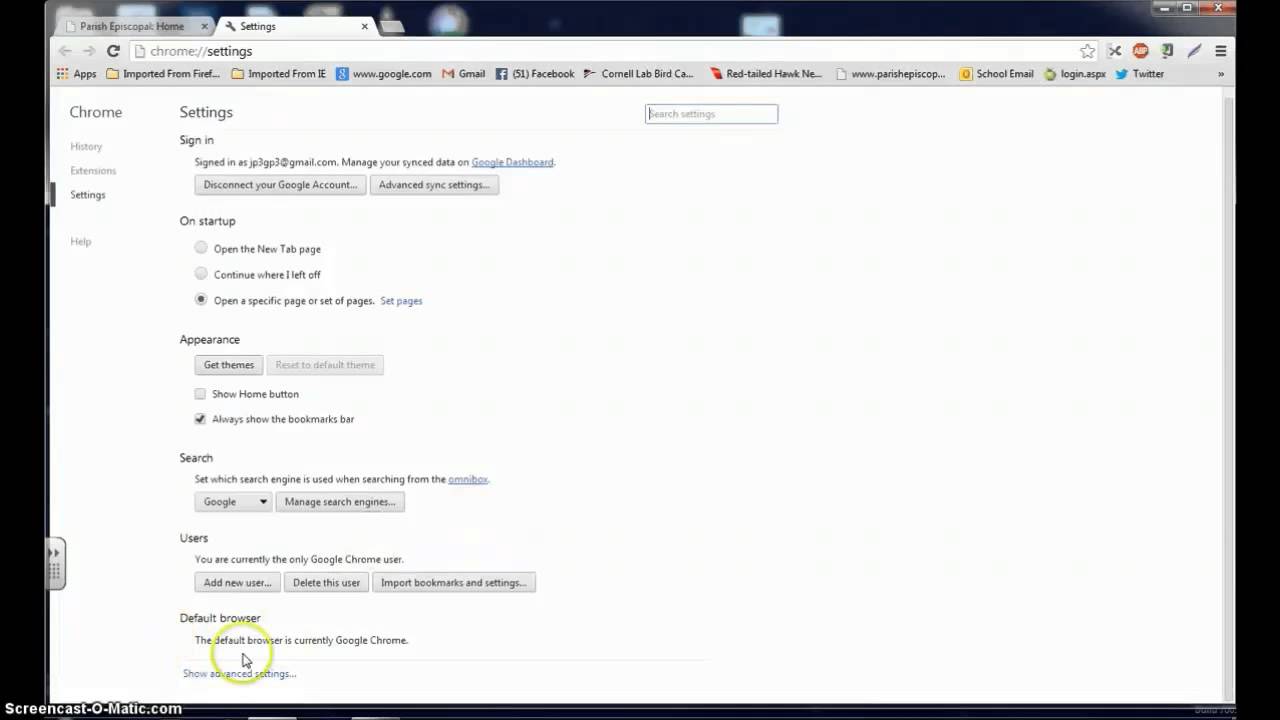This image captures a screenshot of the Chrome web browser with the Settings tab open. In the URL bar, it clearly reads "chrome://settings," indicating that the user is accessing Chrome's settings panel. At the top of the browser window, multiple tabs are open, including one labeled "Path Experiences Home."

The bookmark bar is visible, showcasing several bookmarked websites such as Google.com, Gmail, Facebook, Cornell Lab, and Twitter, along with folders like "Imported from Firefox" and "Imported from IE." The bookmarks indicate a diverse range of interests and frequently visited sites.

The central focus of the settings panel reveals various options available to customize the browser. The user is prompted to sign in, with a partially visible Gmail address. The visible sections include settings for appearance, startup behavior, default search engines, user profiles, and whether Chrome is set as the default browser. The text is relatively small, making some details hard to read, but the overall layout and options of the settings panel are clearly presented.

This detailed screenshot effectively illustrates the typical settings interface within the Chrome web browser, highlighting its functionality and user's customization options.